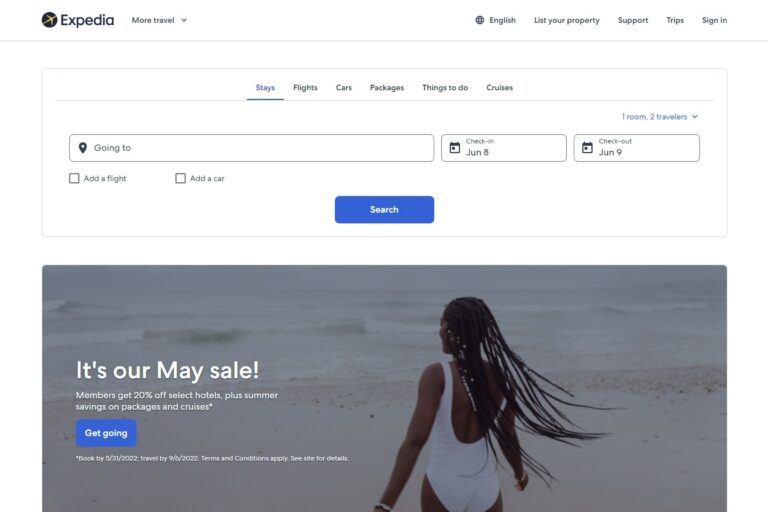The image depicts the homepage of Expedia, characterized by a predominantly white background. At the bottom, a stock photo showcases a black woman walking along the beach with extremely long braids, wearing a white one-piece bathing suit. The image is part of a May sale promotion indicating that Expedia members can enjoy 20% off on selected hotel bookings, along with summer savings on packages and cruises. A prominent blue "Get Going" button is visible underneath the promotional details.

Above the promotional section, the interface presents various travel options: flights, cars, packages, things to do, cruises, and stays. Currently, the user is in the "stays" section, where input fields for the destination, check-in and check-out dates, and additional settings for adding flights or cars are displayed. The user has not entered a destination but the check-in date is set to June 8 and the check-out date is June 9. A blue search button is located next to these fields.

At the very top of the page, there are several links including options to set the language, list a property, access support, view trips, and sign in. The Expedia logo, which features a plane flying through the air, is also visible next to a dropdown menu labeled "More Travel."